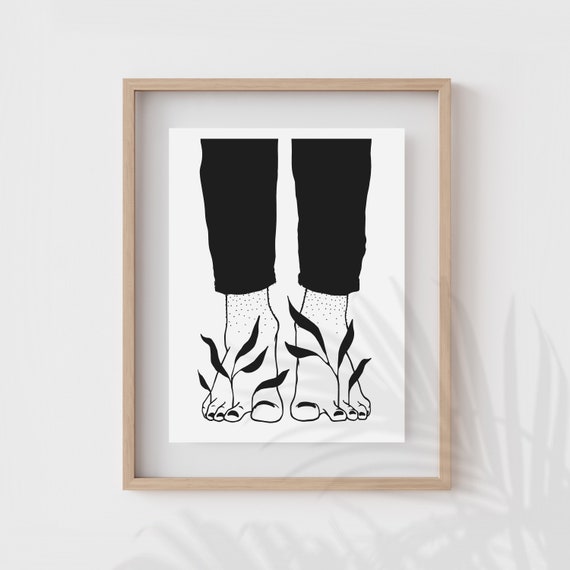This photographic image captures a framed black and white drawing, which is hanging on a light gray wall indoors. The frame is a light brown wood, complemented by a white mat that surrounds the drawing. The artwork within the frame depicts two bare feet protruding from the bottom of a pair of black pants. Intriguingly, small plants appear to be growing between the toes of the feet, with the toenails painted black for added detail. The setting of the print contrasts with its surroundings, possibly suggesting an outdoor scene within an indoor space. A gray watermark, shaped like leaves, is visible in the bottom right-hand corner of the image, subtly blending into the artwork.